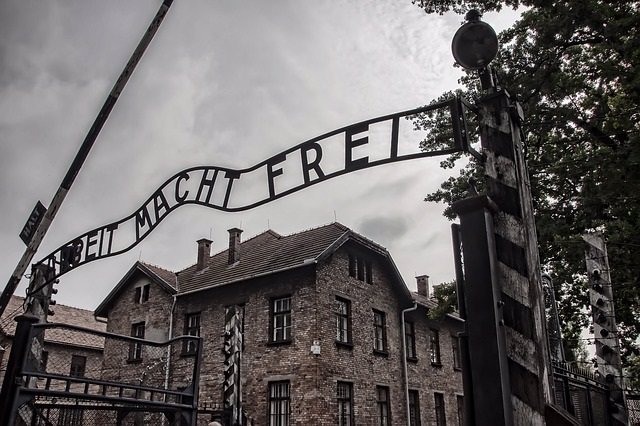The image depicts a somber scene of an old, large brick building adjacent to train tracks, suggestive of an entrance to a former concentration camp, likely Holocaust-related. Black-and-white in composition, the photograph accentuates the gloomy and overcast sky filled with dark, gray clouds. Centered is a horizontal, rectangular metal sign that reads "ARBEIT MACHT FREI," the infamous phrase meaning "Work Sets You Free," a tragic relic of Nazi propaganda. The weathered building features numerous windows—eight on the top floor and eight on the bottom—with an attic space, all displaying years of soot and decay. In the foreground, a railroad crossing lever with striped pole adds to the historic grimness of the scene, underscoring the industrial efficiency of the Holocaust. To the right, a tree partially intrudes into the frame, and on the left, a tall, slim cylindrical pole stands sentinel. This image, a stark black-and-white photograph, freezes in time the haunting entrance, intended to ensure the world's remembrance of one of history's darkest periods.